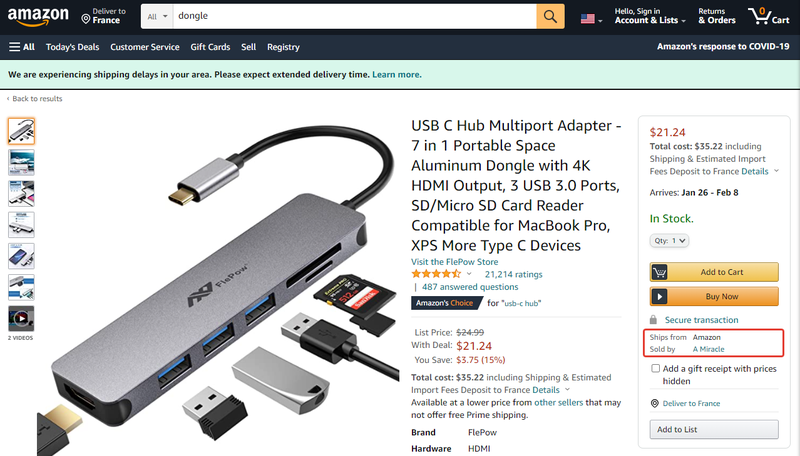This detailed image captures an Amazon webpage with a black header. In the top-left corner, the recognizable "Amazon" logo is displayed in white lettering, complemented by the familiar yellow arrow. Adjacent to this logo is a notification stating "Deliver to France." Below the header is a grey navigation bar featuring options like "Today's Deals," "Customer Service," "Gift Cards," "Sell," "Registry," along with information about Amazon's response to COVID-19.

Situated centrally is a prominent search bar, to its right the American flag icon, followed by account-related options: "Hello, Sign in," "Returns & Orders," and a shopping cart icon, which currently indicates '0' items.

The main focus of the page is the selected product: a "USB-C Hub, Multiport Adapter, 7-in-1 Portable Space Aluminum Dongle with 4K HDMI Output." Accompanying this product listing is an image of the USB-C hub, which features a sleek grey design and a black cable with a USB-C connector attached at the end.